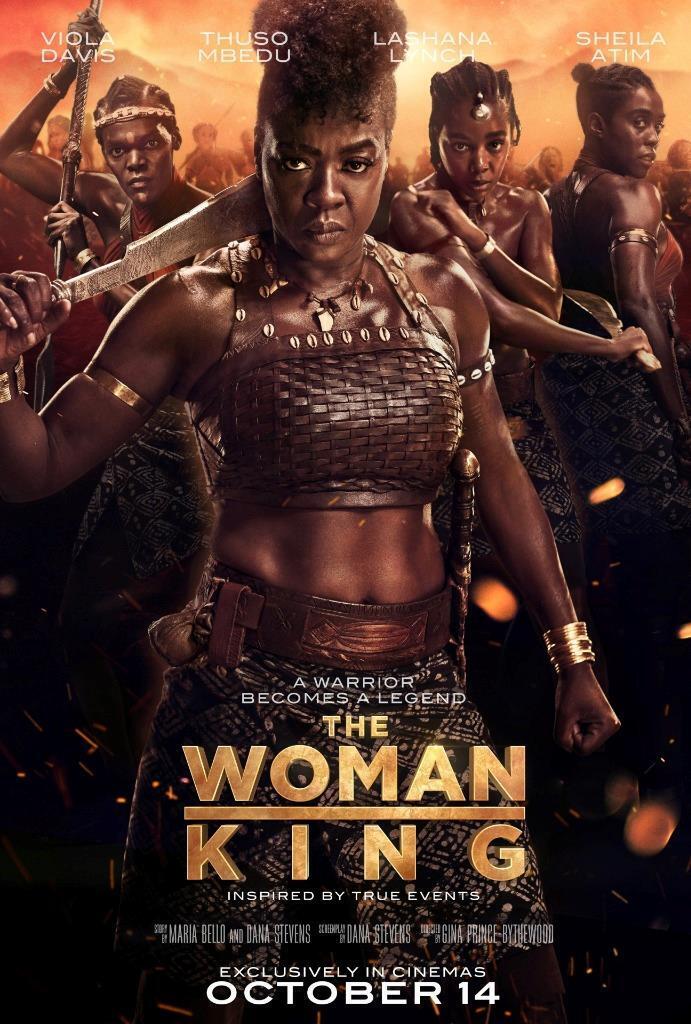The image is a detailed movie poster for "The Woman King," featuring an all-black cast with Viola Davis front and center. She is dressed in dark brown leather warrior garb, comprising a woven crop top adorned with shells, a leather belt, and bottoms that are partly obscured by text. Viola has a serious look, her hair styled into a high poof, and she holds a metal weapon near her neck. Surrounding her are three more fierce black women, each brandishing weapons like swords, knives, or spears, and dressed similarly in warrior attire. The background depicts a fiery, volcanic landscape, adding to the dramatic atmosphere. 

At the top of the poster, the actors' names—Viola Davis, Thuso Mbedu, Lashana Lynch, and Sheila Atim—are written in white text. The tagline "A warrior becomes a legend" is displayed beneath Viola's midsection in white letters, while the movie title, "The Woman King," appears in large goldish-brown lettering below it. Underneath the title, the poster notes that the story is "Inspired by True Events" in smaller white text. Further down, it mentions "Exclusively in Cinemas" with the release date "October 14" in bold, capital letters.